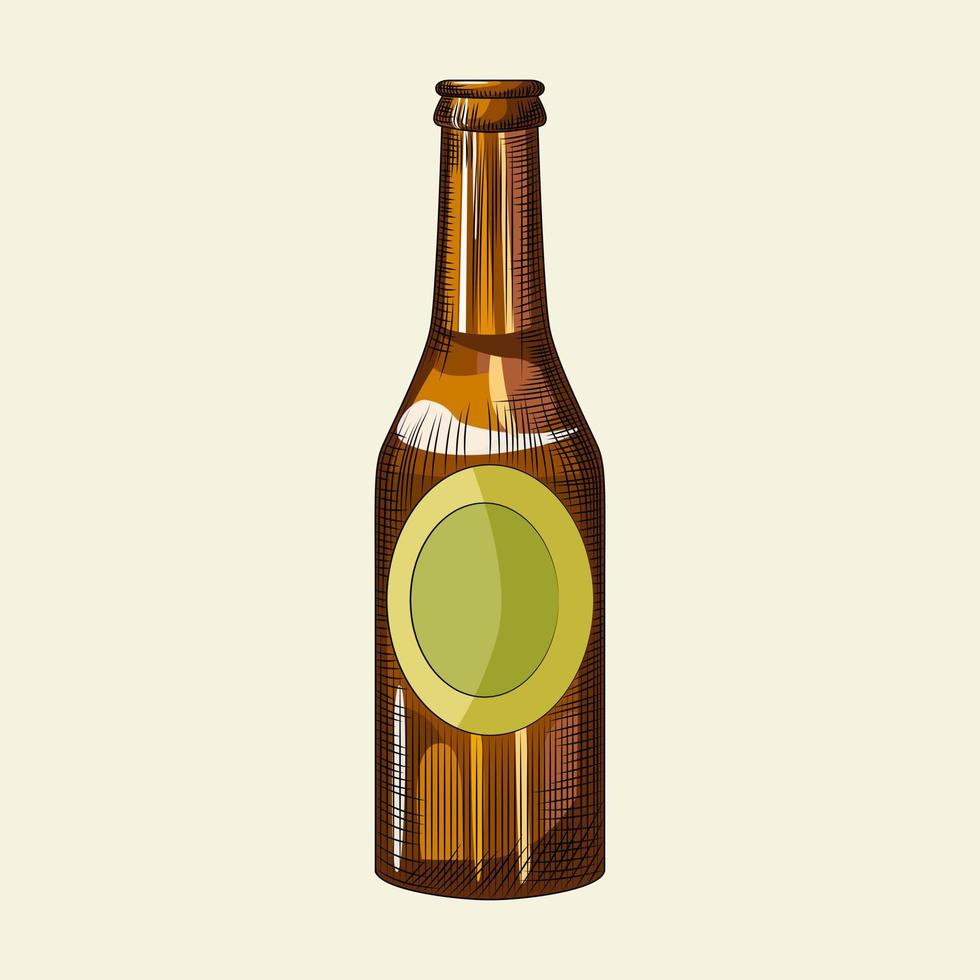The image depicts a digital illustration of a brown glass bottle set against a creamy off-white background. The bottle, rendered with various shades of brown—from dark to light—features intricate crosshatching and curved lines to depict reflections and give a sense of depth and curvature. Its label is composed of two concentric ovals: the outer oval is a medium pea green and the inner oval a darker pea green, with both bordered by a black oval. Despite the simplicity of the overall design, the proportions are professional, and the bottle's details, including its neck and opening, are accurately portrayed. The absence of text on the label and the minimalistic background further highlight the bottle's form.